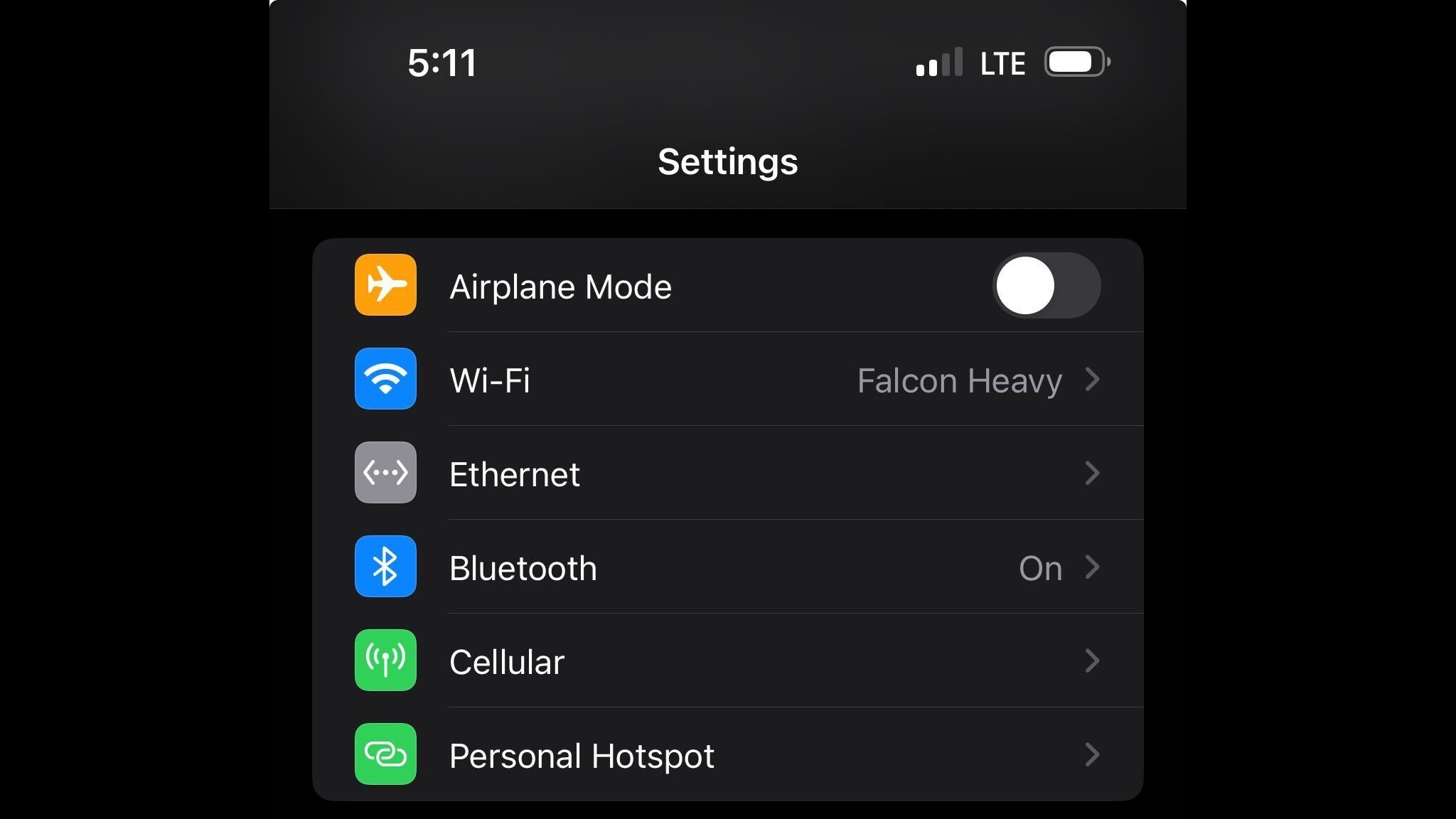A detailed and cleaned-up caption for the provided description of the image could be:

"This image is a screen capture from a mobile device, most likely an iPhone. The time displayed at the top center reads 5:11, while the top right corner shows LTE connectivity, a battery icon, and a Wi-Fi signal strength indicator. Below these status icons, the screen indicates that the user is viewing the 'Settings' menu, with options including 'Airplane Mode' (switched off), 'Wi-Fi,' 'Ethernet,' 'Bluetooth,' 'Cellular,' and 'Personal Hotspot.' The background color of the screen capture is predominantly black, with the settings menu displayed in a very dark gray hue."